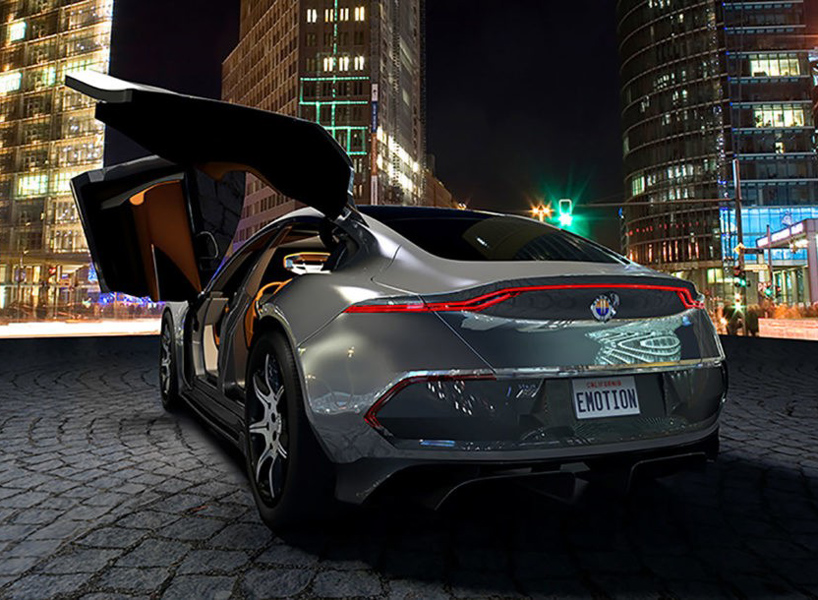This is a horizontal rectangular image capturing the rear view of a sleek, foreign-made luxury sedan parked on a cobblestone street in a city at night. The car, painted in a shimmering silver-gray hue, features stylish gull-wing doors—one open vertically on the passenger side and one ajar at an angle. The vehicle’s large wheels are adorned with chrome trimming and silver rims, while the windows are tinted black, with a beige interior subtly visible. Prominently displayed on the car’s license plate is the word "Emotion." The background reveals an urban nightscape bathed in artificial light: three tall buildings with illuminated windows, and a bright green streetlight casting a glow over the scene. The image is detailed with reflections in nearby windows and the artistic quality of a city alive at night.